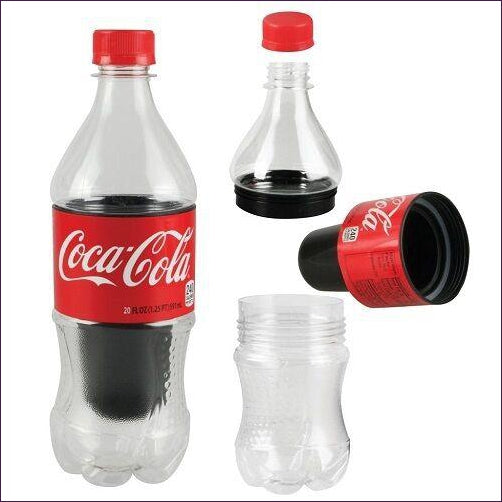In a square image with a small black border and a white background, we see two Coca-Cola bottles made of plastic. The bottle on the left is fully assembled, featuring a red label with white "Coca-Cola" text and a red cap. Visible through the transparent bottle is an inner black structure, possibly a filter or a cup, that runs from just below the cap to about an inch above the base.

The bottle on the right is disassembled into four distinct parts: the red cap, the clear top portion, the middle section with the red label and the black inner cup, and the clear base. This inner black cup or filter can be removed by unscrewing the top and bottom sections of the bottle. The image appears to be showcasing a novelty or decoy bottle that, when fully assembled, looks like a standard Coca-Cola bottle with an unusual internal compartment.